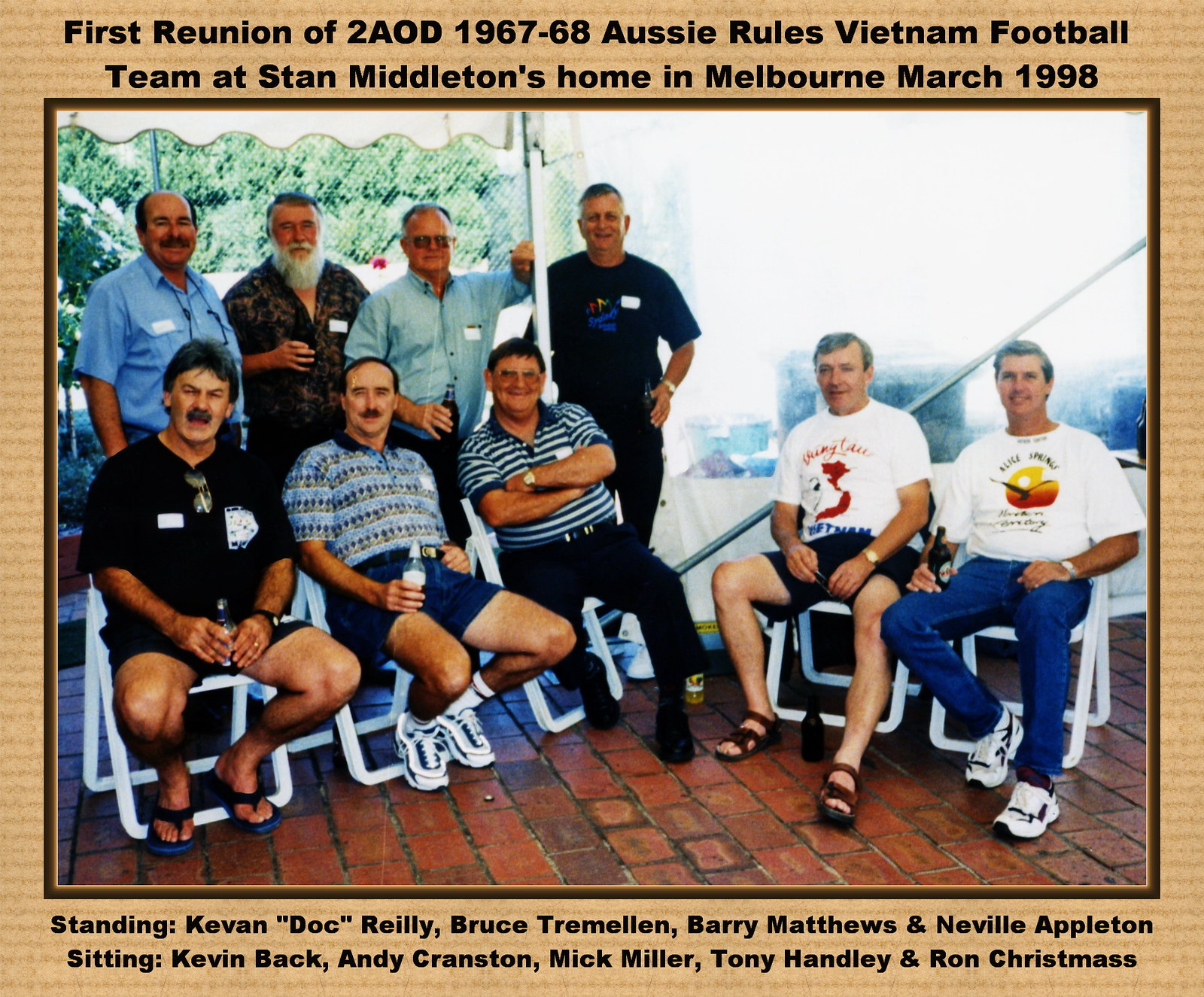The image captures the first reunion of the 2AOD 1967-68 Aussie Rules Vietnam Football Team, held at Stan Middleton's home in Melbourne in March 1998. In the photo, nine team members are present: four standing in the background and five sitting in the foreground on white folding chairs over a red brick ground. The caption at the top of the image reads, "First Reunion of 2AOD 1967-68 Aussie Rules Vietnam Football Team at Stan Middleton's home in Melbourne, March 1998." In black font below the image are the names of the men, with the standing members being Kevin "Doc" Riley, Bruce Tremellin, Barry Matthews, and Neville Appleton. The seated members are Kevin Back, Andy Cranston, Mick Miller, Tony Hanley, and Ron Christmas. 

The photograph features men dressed in casual attire, clearly enjoying each other's company. Specific details include two men on the left wearing white t-shirts with symbols on the front, one of whom has blue jeans and white running shoes, while the other is in shorts and flip flops. Among the standing men: one is bald with a mustache and wears a blue shirt; another sports a dark brown and black shirt with a long gray beard; a third holds a beer and wears a light blue shirt; the fourth has a black t-shirt with a central symbol. The scene illustrates a significant gathering, celebrating the 30-year reunion of these former teammates.